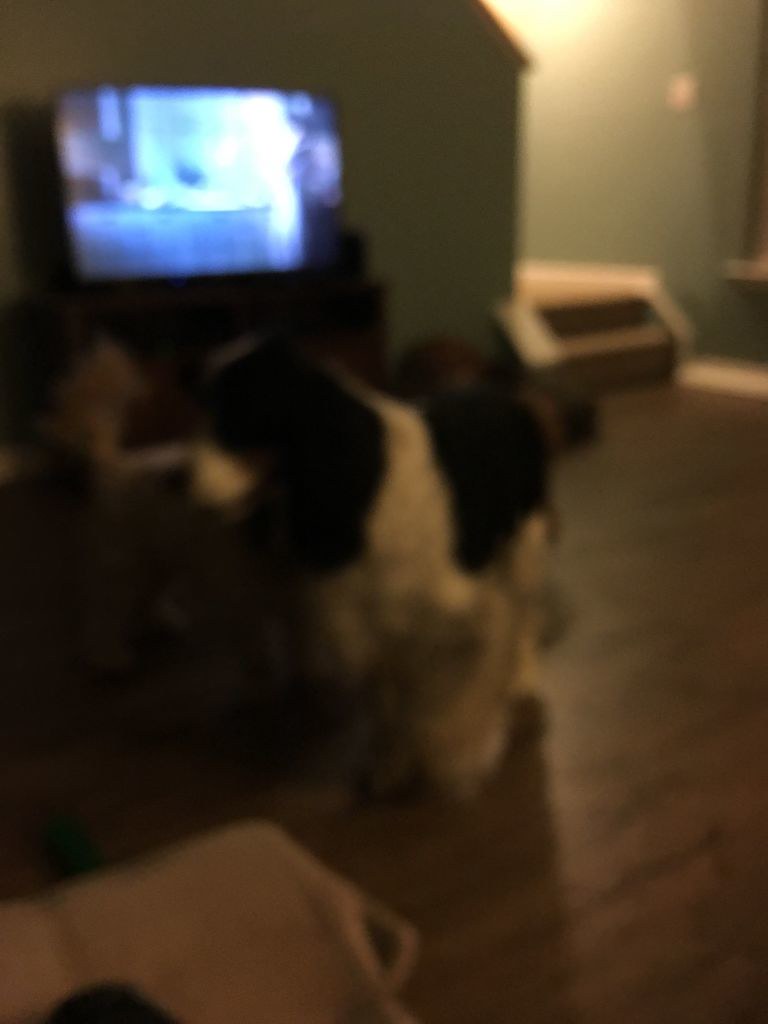This is an image taken inside someone's home, though it is significantly blurred and distorted, making details hard to discern. The lower portion features what seem to be hardwood floors or dark laminated wood floors. In the background, there's a blurred staircase ascending, bordered by walls that are either teal or celery green. The image also reveals a railing and a light switch, indicating a standard interior layout with multiple rooms. A TV or computer monitor is vaguely visible amid the blurriness, possibly nestled in a credenza or cabinet.

In the foreground, a person appears to be holding or petting a dog. The dog has distinct coloring: it has black, fluffy ears, a white body with areas of dark brown around its head, neck, and back, and white down its front and on its feet. The scene includes part of a chair, potentially with a beige cover, and suggests another small dog may be present. There is also a white item, possibly a bag or backpack, hanging from the chair. The complex interplay of objects and colors, though difficult to fully clarify, hints at the warmth and activity typical of a lived-in home.